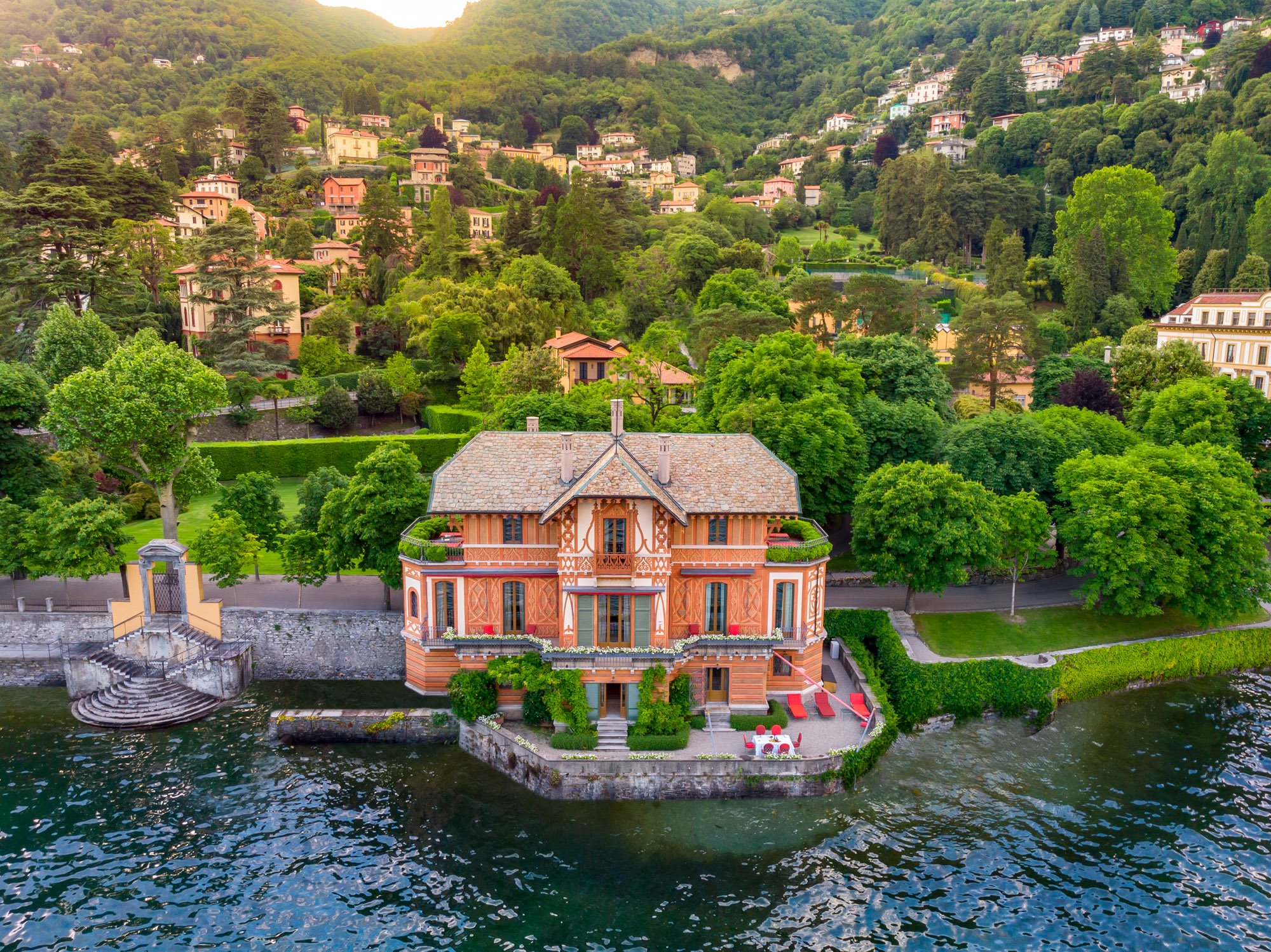This detailed photograph showcases a grand, three-story, reddish-orange brick mansion situated prominently along the edge of a serene body of water, possibly a lake or river. The mansion's distinctive features include tall, floor-to-ceiling paned windows that offer expansive views of the water, and a more brownish-gray, eaved roof. Setting the scene, a lush, green landscape with numerous deciduous trees surrounds the mansion, and a road or biking path runs behind it. Many similarly colored homes, with a cohesive palette of peach and terracotta hues, dot the hillside in the background, suggesting a picturesque European village.

The mansion itself is built on an elevated stone pier that extends into the water, enhancing its stately presence. A notable outdoor patio near the water features a dining table adorned with a white tablecloth and surrounded by six red chairs, perfect for alfresco meals. Adjacent to this is a set of three red lounge chairs, inviting relaxation by the water's edge. Adding to the charm and functionality, a cascading staircase on the mansion's left side leads directly down to the water, where residents could conveniently access a boat. The sun is visible in the top left corner of the image, casting a warm, inviting glow over the entire scene.